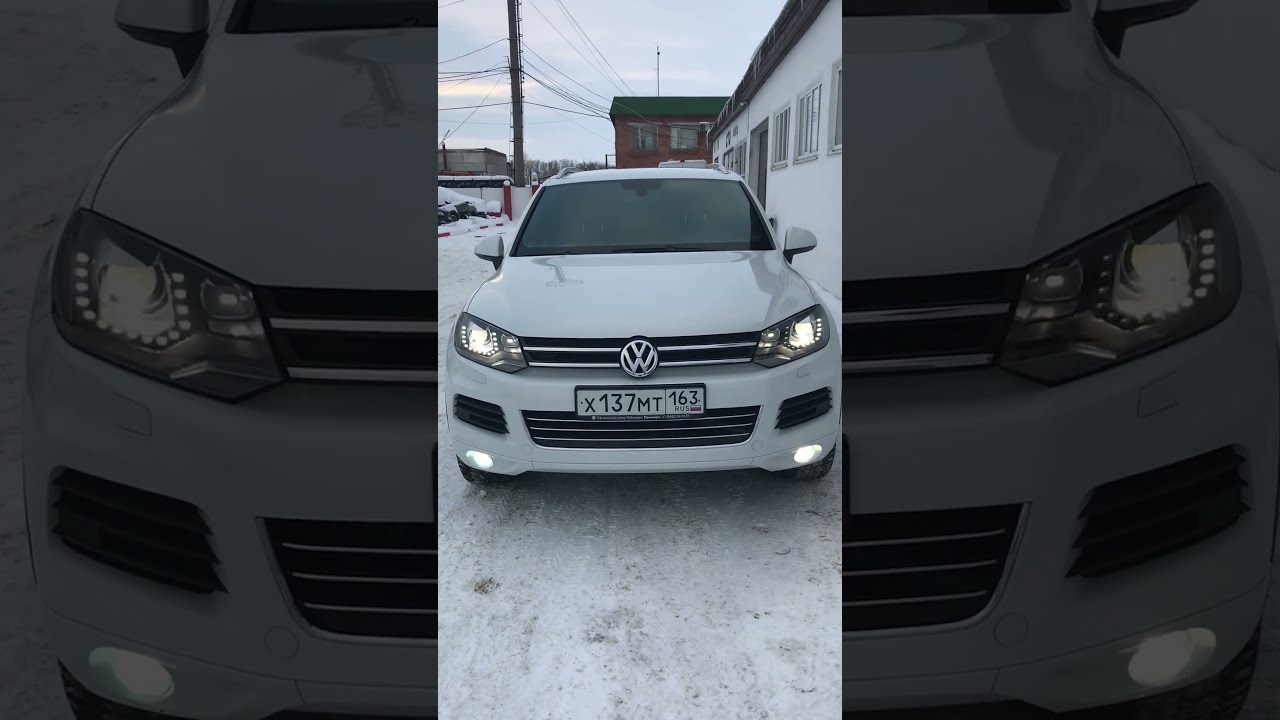This image captures a light silver, newer model Volkswagen car with black trim and its headlights turned on, prominently displaying a European style license plate with the number X137MT163. The car is positioned centrally on a road surface, which appears to be either lightly snow-covered or covered in white dirt, amidst a wintery, cloudy daylight setting. The backdrop includes a white building with several windows and doors to the right, a brick red building with a green roof to the left, and a telephone pole. The sky is overcast with dense clouds and power lines can be seen in the upper left corner. No people are visible, focusing attention entirely on the car and the surrounding environment.